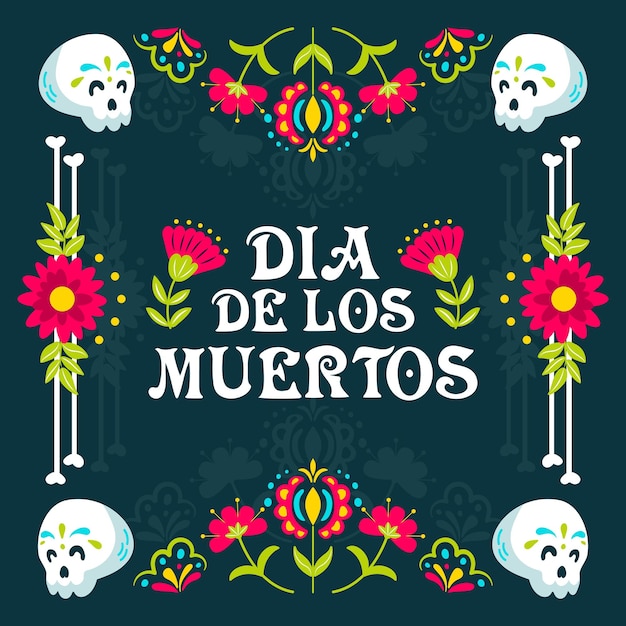The image resembles a vibrant greeting card, bordered by a black rectangular background. Each corner of the card features a cartoon-like white skull, adorned with green and yellow painted blobs in the positions of eyebrows. Between the skulls are clusters of red and yellow flowers with lush green leaves. On the left and right sides of the image, extending towards the skulls, are cartoon-like bones interspersed with additional flower designs. The card is rich with floral patterns, some of which are shadowed to add depth to the background. 

At the center, the phrase "Día de los Muertos" is elegantly written in white font, flanked by two red and green flowers on either side, enhancing the festive feel of the design. This greeting card beautifully combines whimsical skulls, bones, and vibrant floral motifs to celebrate the Day of the Dead.